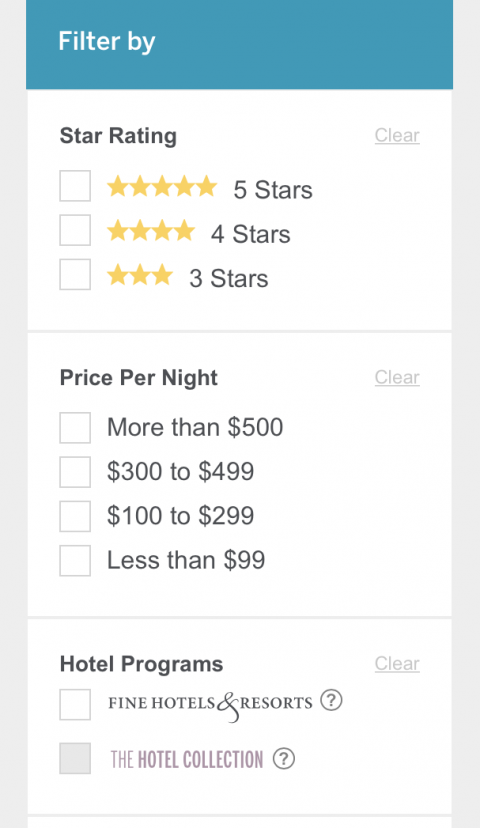The image features a user interface for filtering search results on a light blue background. At the top, there is a dark blue box with the text "Filter by" in white. Below it, a white section is dedicated to filtering by star rating. This section includes individual boxes for different star levels: 
- Five stars
- Four stars
- Three stars

In the top-right corner of this section, there is an underlined "Clear" button for resetting the filters. 

Separating the star rating filter from the next section is a horizontal line. The subsequent section is labeled "Price per Night" and contains boxes for various price ranges:
- More than $500
- $300 to $499
- $100 to $299
- Less than $99

This section also includes an underlined "Clear" button. 

Another horizontal line separates the price filter from the next category, "Hotel Programs." Here, there is a box labeled "Find Hotels and Resorts," alongside a circular icon with a question mark. To the right of this box is another underlined "Clear" button. Beneath it, a blue box labeled "The Hotel Collection" includes another circular icon with a question mark.